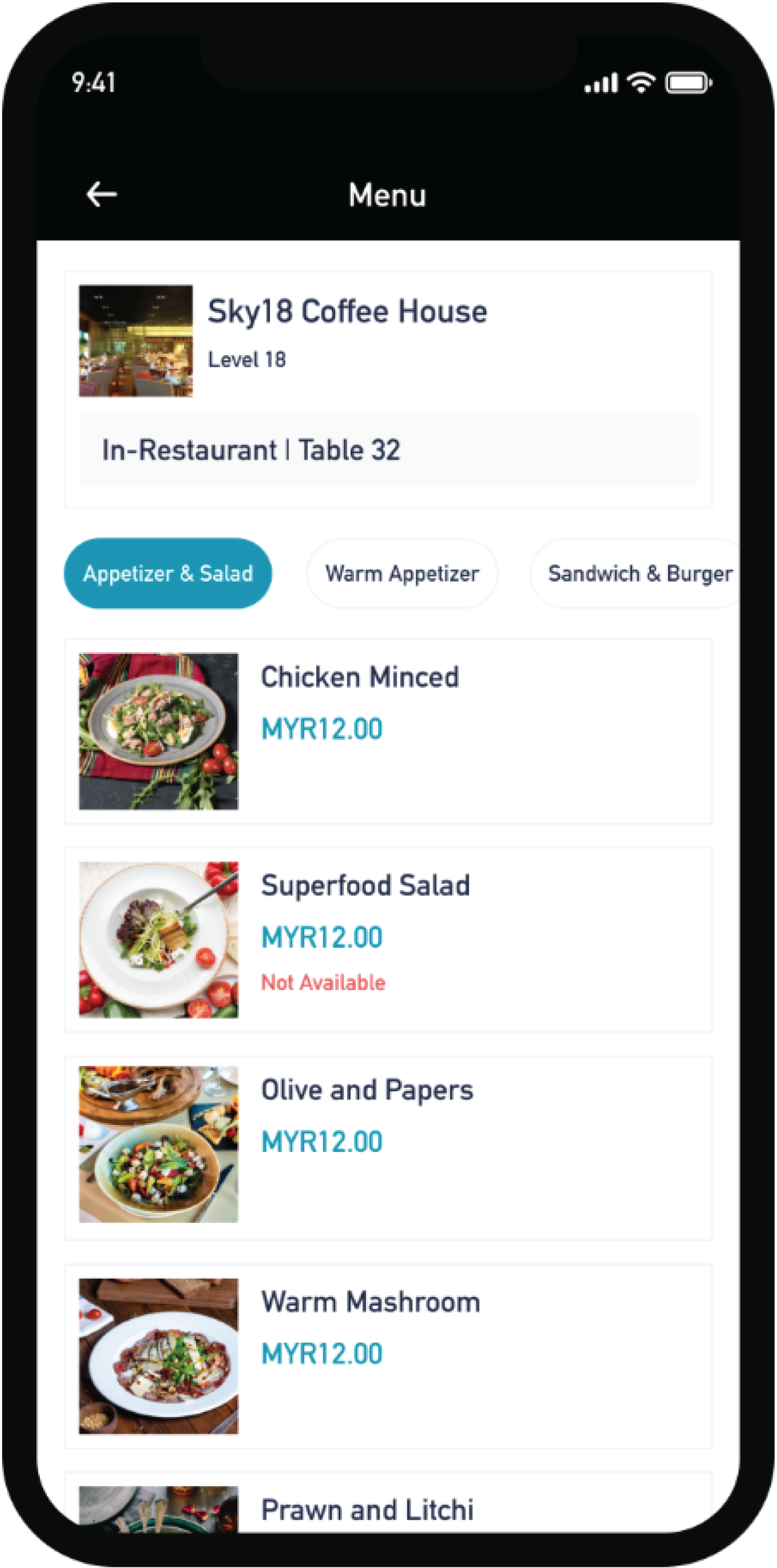The image is a screenshot depicting a digital menu interface of a restaurant, likely viewed on a mobile device. At the top right corner of the image, the status bar shows a fully charged battery icon, a full Wi-Fi signal indicator, and a full phone signal strength icon, sequentially from right to left. On the top left, the current time is displayed as 9:41. Positioned centrally at the top of the screen is the word "Menu," with a white leftward-pointing arrow immediately to its left.

Below this header, the name of the restaurant, "Sky 18 Coffeehouse," is prominently displayed, along with its location on "Level 18." Adjacent to the restaurant name, on the left side, is a small squared box featuring an image of the restaurant. 

Immediately below, there are three category bubbles designed to help navigate the menu: "Appetizer and Salad" in a blue bubble, "Warm Appetizer" to its right, and "Sandwich and Burger" further right. 

Further down, specific menu items are listed: "Chicken Minced," "Super Food Salad," "Olive and Peppers," "One Mushroom," and "Prawn and Lychee."